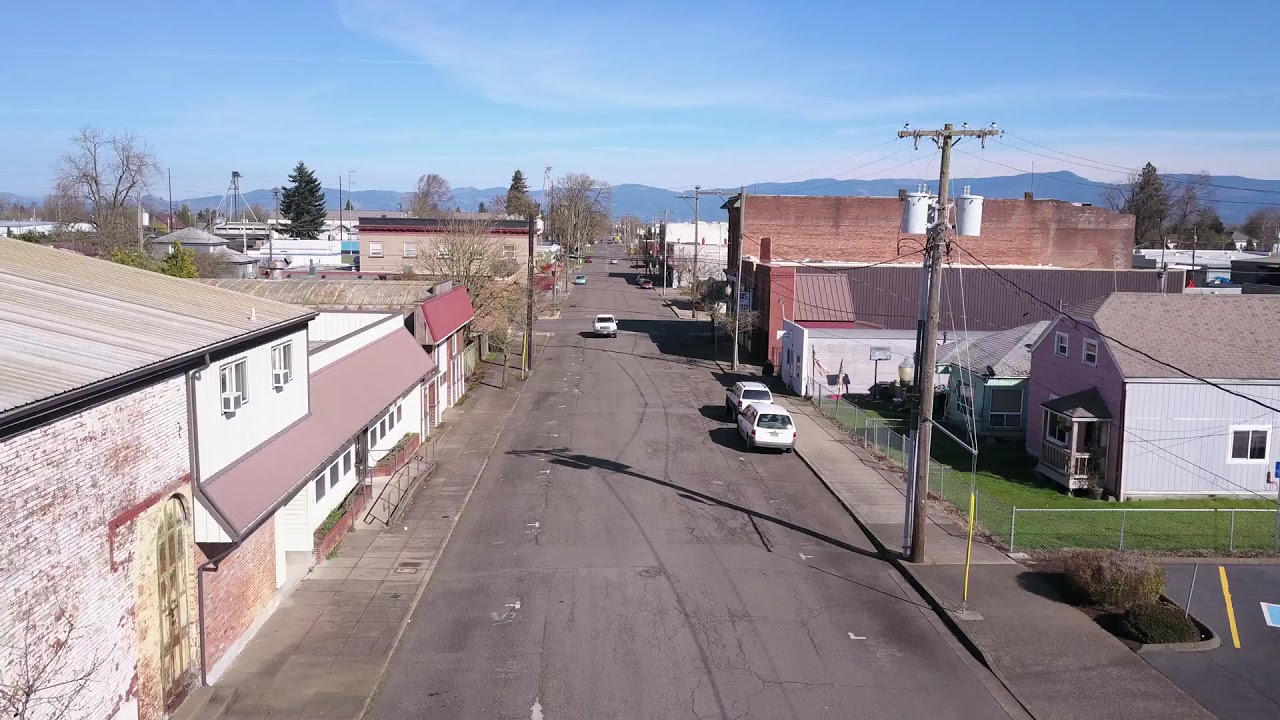In this brightly lit photograph taken on a sunny day, we are presented with a vivid scene of an old town's main street, viewed from a high vantage point, possibly a drone. The street runs straight up the center of the image, stretching into the horizon where a faint mountain range meets a bright blue sky adorned with wispy clouds and a touch of pink. This two-way, blacktop road features sectioned-off, white parking spots on both sides, with two white cars parked on the right and another white car driving towards the camera on the left.

Flanking the street are wide sidewalks lined with power lines and various buildings. On the right side, these include a mix of houses and square, brick buildings. The left side showcases a blend of brick and weathered shopping buildings, their white paint peeling, adding to the rustic charm. Notably, a large, connected factory-type building dominates the left, accompanied by small shops. The scene captures the essence of a serene, less-frequented old American town, encapsulating its antiquated, boxy architecture within a picturesque urban landscape.